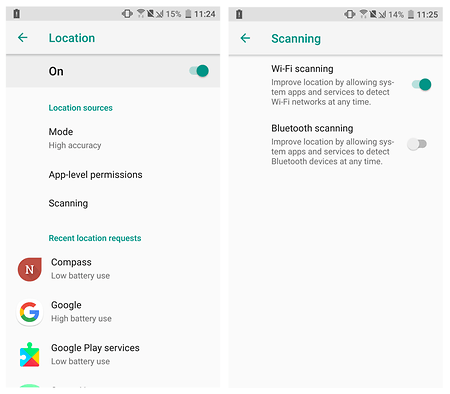The image comprises two side-by-side screenshots captured from a mobile device, each showcasing different functions. The left screenshot focuses on location settings, with the top portion featuring the word "Location" in green text, accompanied by a green arrow pointing left, indicating a back navigation option. Below this, it is indicated that location services are enabled ("on"). Further down, it displays "Location Sources" in green, followed by additional detailed options not fully visible in the screenshot. At the bottom of this screen, the Google Play Services logo is present, depicted as a colorful jigsaw puzzle piece in shades of green, red, yellow, and blue.

The right screenshot emphasizes scanning features, starting with the word "Scanning" in green text at the top, paired with a green arrow also pointing left for back navigation. Directly underneath, it lists "Wi-Fi Scanning" with an associated toggle button to the right, which is switched on, signifying that Wi-Fi scanning is currently active. The visual layout of this screen is more simplified compared to the left, focusing primarily on the scanning options available.